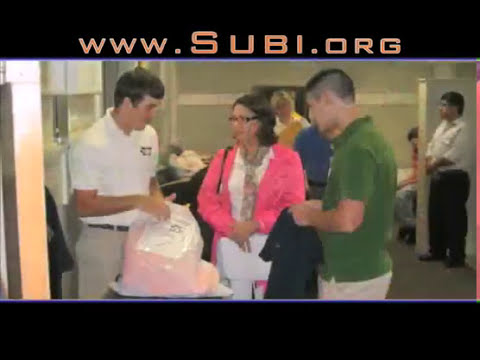The image is an advertisement featuring a website URL, www.subi.org, displayed in orange text on a black background at the top. The main photograph showcases a business casual scene inside what appears to be a hotel or conference room, with a black bar at the bottom edge mirroring the one at the top. In the center of the image are three people. On the left stands a man with short brown hair, dressed in a white polo shirt, khaki pants, and a brown belt. He is holding what seems to be a white plastic bag and is gazing towards the others. In the middle, a woman with short brown hair, glasses, and a hot pink cardigan over a white blouse looks towards the white-shirted man. To her right, another man with buzzed dark hair, wearing a green short-sleeve polo shirt and khaki pants, holds a piece of black clothing while also looking at the man in the white shirt. The setting includes a few indistinct figures in the background, contributing to the overall sense of being in a communal or professional environment.